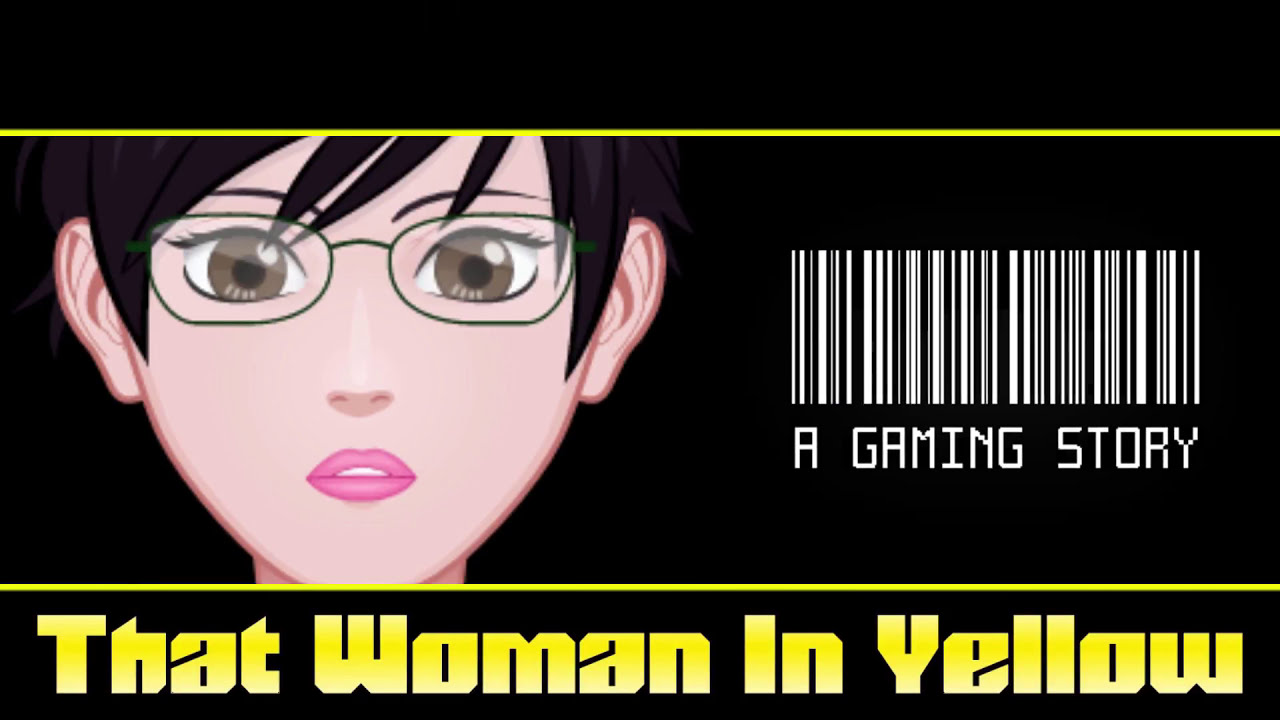The image is a computer-generated, anime-inspired graphical design featuring a close-up of a woman's face on the right side, staring forward. The woman has peach-colored skin, large brown eyes with white reflective spots, and distinctive green-rimmed glasses that extend behind her short, black hair, which falls just to the level of her ears. Several strands of hair reach down to the level of her eyes, just below her eyebrows. Her lips are vividly pink, resembling pink lipstick, and her small nose is white. The image is framed by thin yellow bars at the top and bottom. The bottom bar includes uppercase yellow text that reads "THAT WOMAN IN YELLOW". To the right of the woman’s face, there's a white barcode followed by the text "A GAMING STORY" in white uppercase letters. The background surrounding the design is black, with the yellow elements providing a stark contrast.